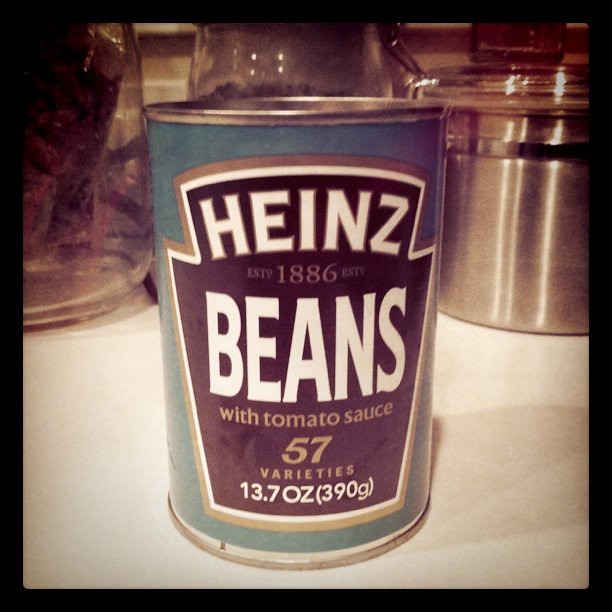The square image prominently features a blue can of Heinz Beans placed on a pristine white countertop. In the background, there are three jars: a stainless steel jar on the back right and two glass jars positioned in the middle and back left. The can of Heinz Beans, adorned with a distinct shape, stands out with its bold white text displaying "Heinz Beans." Between "Heinz" and "Beans," the can details "EST. 1886." Below "Beans," in yellow text, it reads "with tomato sauce, 57 varieties," followed by "13.7 ounces (390 grams)" in white text.